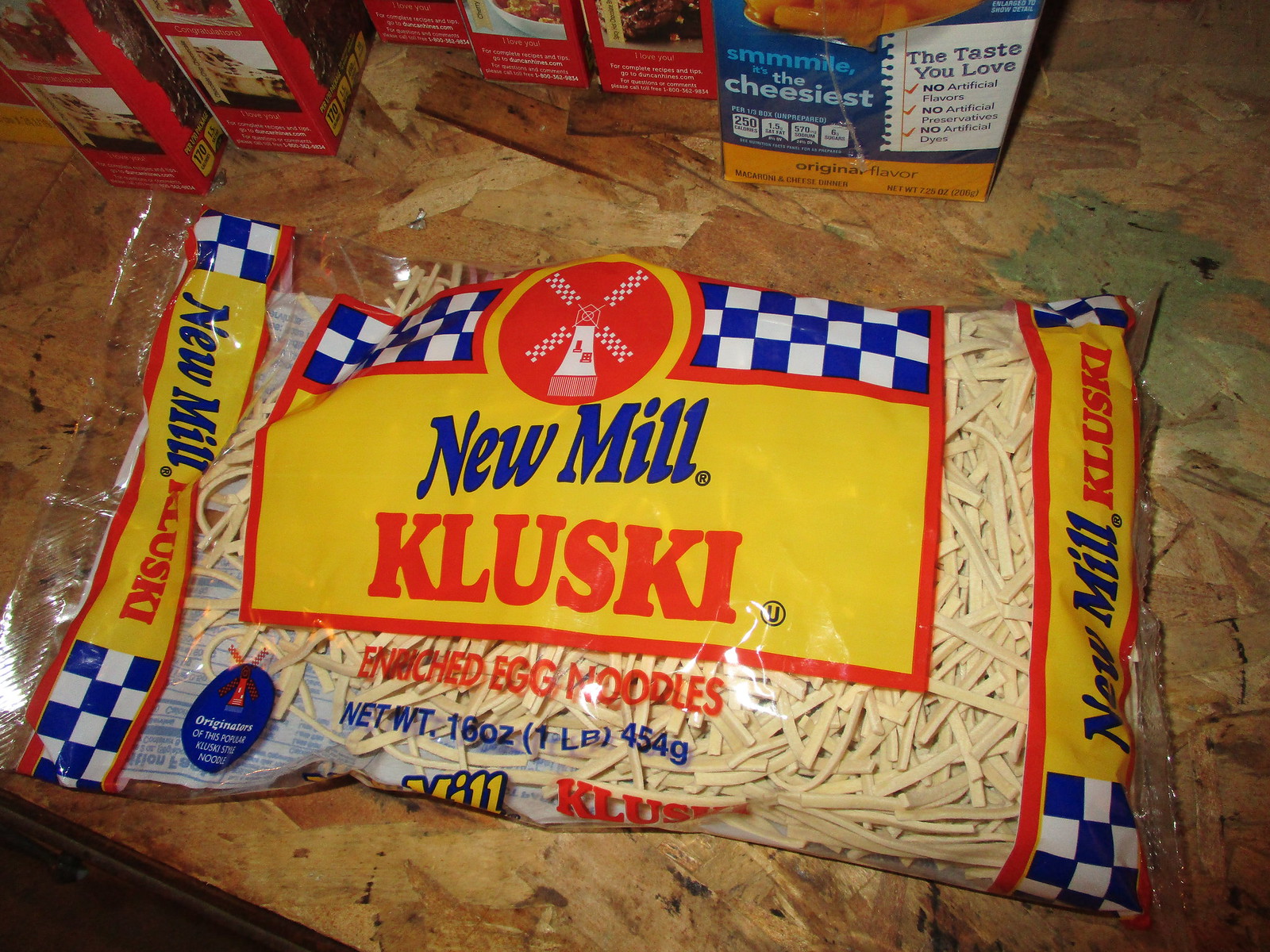The image showcases various food products displayed on a plywood surface. Five boxes are arranged in the background with their end panels visible at the bottom. One of the boxes is turned backward, revealing a small section of its front with a recognizable blue label featuring an orange border and the text, "Original Flavor, Smile, the Cheesiest," suggesting it's a box of mac and cheese. 

In the foreground, the primary focus is on a bag of noodles laid flat on the table. The packaging prominently reads, "New Mill Kluski Enriched Egg Noodles" with a net weight of 18 ounces. The bag's label is predominantly yellow, featuring a distinctive blue checkerboard pattern at the top, enclosed by a red border. Within the blue checkerboard, there's a red circle containing a white windmill icon. Labels at both ends of the product also state "New Mill Kluski," utilizing yellow with both blue and red print for additional detail and branding consistency.